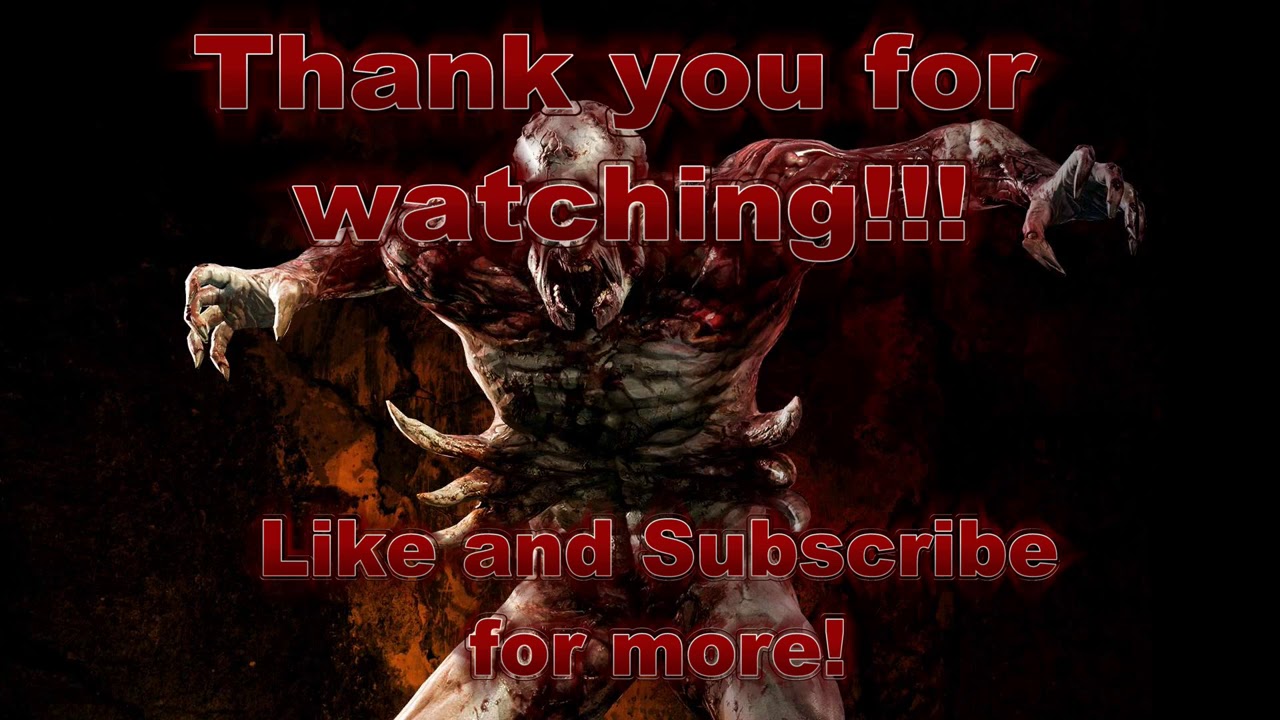The image is a horizontal rectangle with a mostly black background. At the center, there appears to be a brownish, cave-like entrance, where a terrifying, demonic creature stands menacingly. The monster has a grotesque, red and gray scaly body, a bald head, and sharp, human-like claws with elongated fingernails. Notably, two pointy, horn-like protrusions jut out from either side of its waist. The creature's mouth is wide open, appearing to scream, and its arms are outstretched to its sides in a flailing posture. Covering part of the creature's face, red text outlined in white reads, "Thank you for watching!!!" Below this, in the same styled text, it says, "Like and subscribe for more!" The monstrous figure and the sinister dark background intensify the eerie, high-definition image, creating a scene that is both frightening and arresting.